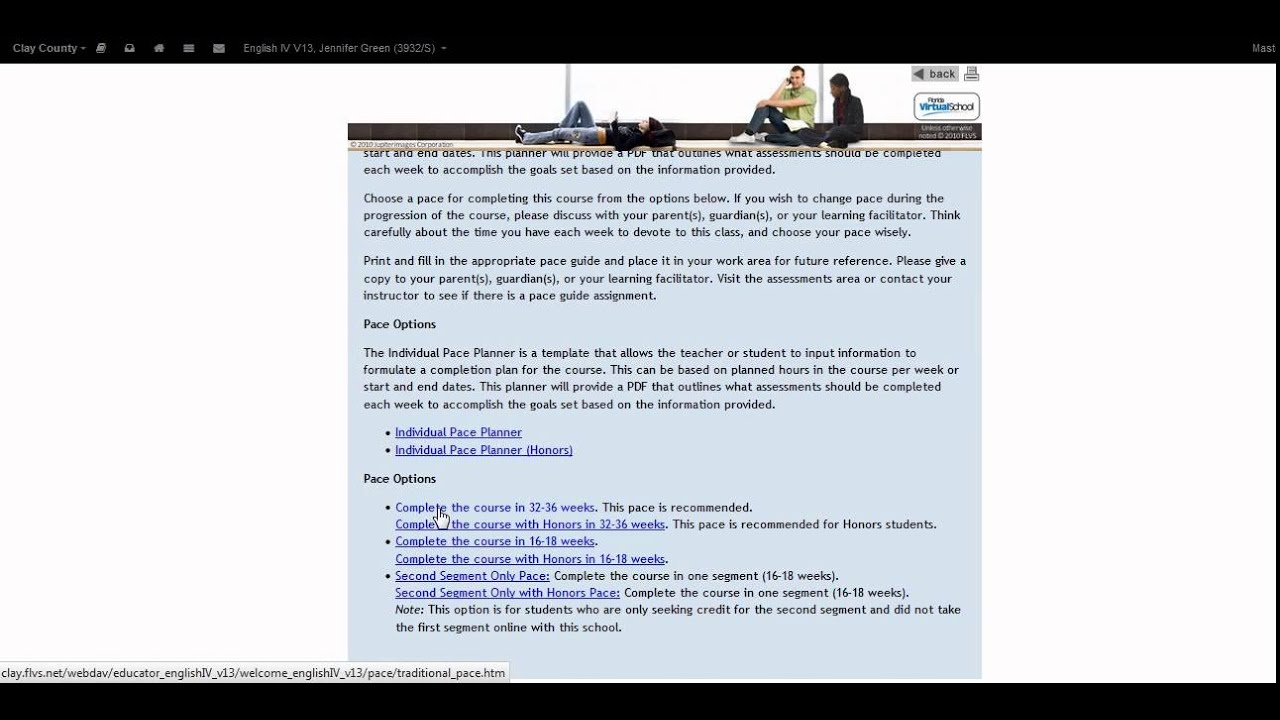This screenshot captures a web page from Clay County. At the top, there is a black navigation bar with white text that reads "Clay County," followed by five small white symbols. Next to these symbols, it indicates "English 5 4 13 Jennifer Green 3 2 or 3 9 3 2/s".

The main body of the web page features images and text. The first row includes three photographs of individuals. The first image shows a girl lying down, wearing jeans and a black shirt, seemingly looking at her phone. The second image is of a man in a green shirt and blue jeans, also engaged with his phone. The third image depicts another man with black hair sitting next to the man in the green shirt.

Below the images, there are multiple paragraphs of text primarily written in black. Certain sections are highlighted in blue, indicating clickable links. On the bottom left-hand side, a very long web address is displayed.

Additionally, at the top right-hand side, near the images, there are icons and options including a back button, a printer icon, and a clickable link for "Virtual School," with "Virtual" highlighted in blue.